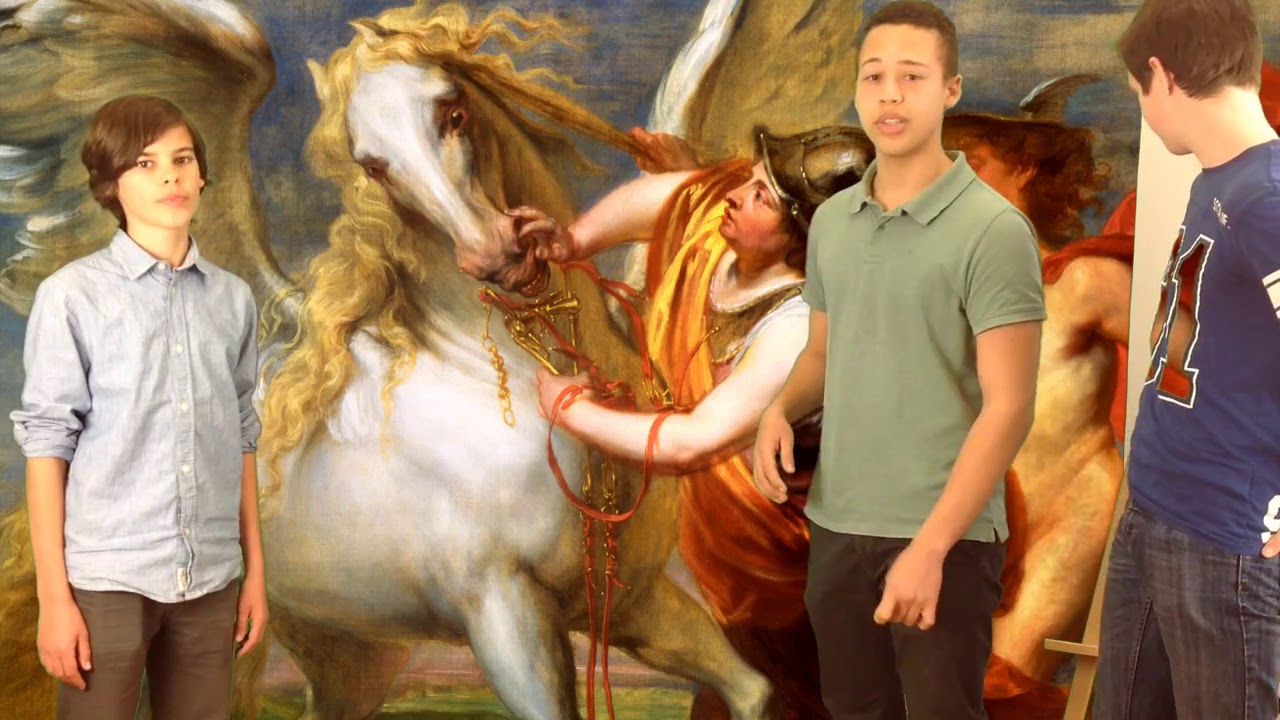In this detailed photograph, three young boys stand in front of an expansive painting that fills the entire background. The painting itself portrays a dramatic scene, where on the left side, a white horse with a golden mane, depicted with wings like a Pegasus, is resisting as a figure attempts to place a bit into its mouth. This figure, wearing a copper helmet and an orange sash, has brown-colored reins draped over their arm. On the right side of the painting, another unclothed figure is assisting, identifiable by a distinctive hat adorned with a wing.

Of the three boys in the foreground, the one on the left stands still with his arms hanging by his sides. He has brown hair covering his forehead and ears, brown eyes, and is dressed in a blue button-up shirt with rolled-up sleeves and brown pants. The middle boy wears a green-collared t-shirt and black pants, characterized by his darker complexion, curly black hair, and brown eyes. He has one hand near his hip and the other slightly raised to the level of his stomach. The boy on the far right has fair skin and light brown hair, visible light reflecting off the back of his neck as he looks backward at the painting's unclothed figure. He sports a blue jersey with a visible number one on it and blue pants with white streaks.